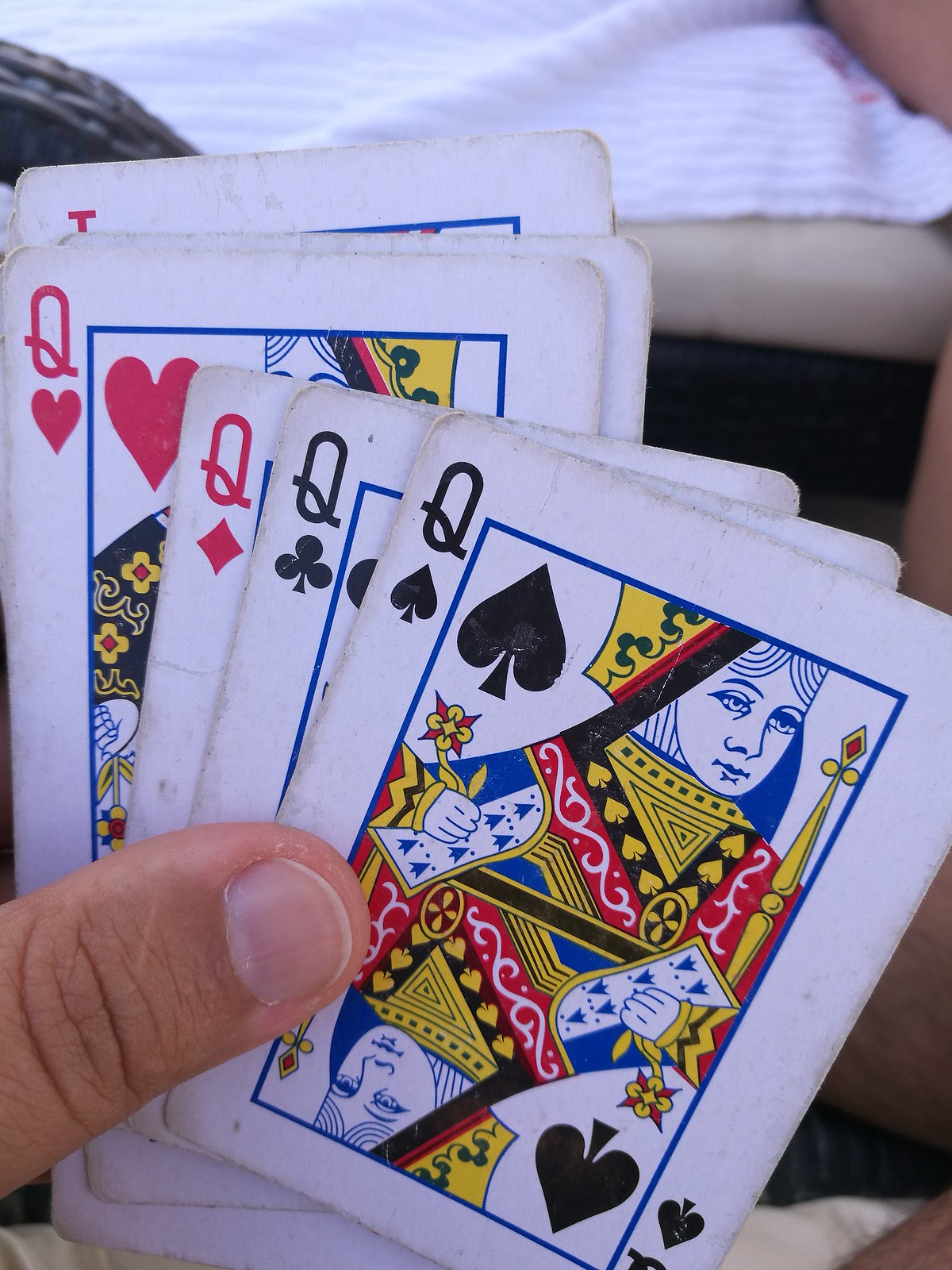In the image, a person is holding a hand of six well-worn playing cards. Prominently displayed are all four queens, with the black queens (spades and clubs) positioned towards the front and the red queens (hearts and diamonds) just behind them. A jack is also visible near the back of the hand, though the identity of the sixth card remains hidden. The scene is set on a light beige tabletop with a small black space underneath, and draped over the table is a towel featuring blue and white stripes. The person's other arm rests upon the table, creating a casual and contemplative atmosphere. The cards show signs of extensive use, with slightly ragged edges and bent corners. The background, once white, now bears the marks of many games played. The individual appears to be puzzling over their hand, considering their next move.